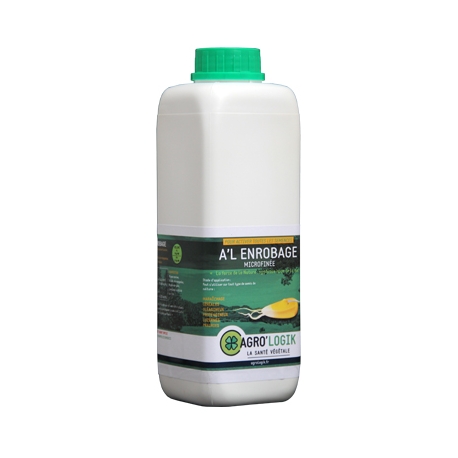The image depicts a white, vertically-oriented, rectangular canister with a rounded-off, cuboid shape on a plain white background. The canister is approximately one quart in size and features a twist-off green cap. Its label, bordered by thin stripes (white at the top and black at the bottom) and thicker reversed stripes (black at the top and white at the bottom), is primarily green. The label includes white capital letters reading "L' E-N-R-O-B-A-G-E," indicating the product or company name. Below this text is an intricate scene: a horizontally-positioned corn kernel to the right and white, jellyfish-like tentacles extending from the left. The label also contains "H-O-C-R-D" in green lettering and "A-G-R-O" in black lettering at the bottom.